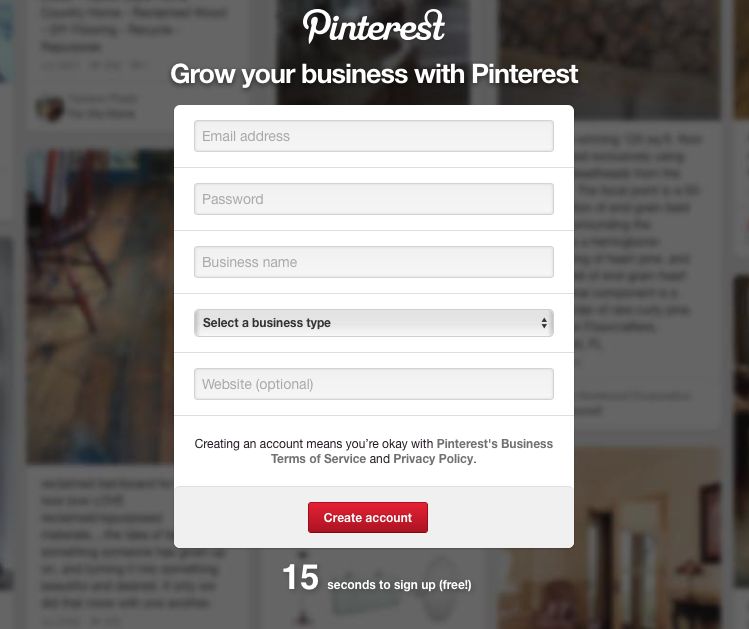The image features a Pinterest registration overlay, designed to create a business account. The interface is constructed with a semi-transparent gray overlay that partially obscures a faint background. The visible portion of the background seems to showcase Pinterest posts, resembling images pinned on a virtual wall, each accompanied by some text above and below.

Central to the overlay, the heading "Grow your business with Pinterest" is prominently displayed in white text. Below this, a white box hosts input fields for "Email address," "Password," "Business name," and a dropdown menu labeled "Select a business type." These fields are pre-filled with gray placeholder text, except for the dropdown menu, which is more distinct. Additionally, an optional field titled "Website (optional)" appears in parentheses underneath the dropdown menu.

At the bottom of the form, a disclaimer reads: "Creating an account means you agree to Pinterest's Business Terms of Service and Privacy Policy," presented in black text. Following the disclaimer is a red "Create account" button with white text, encouraging user action. Adjacent to this, another inscription in white text reads: "15 seconds to sign up (free)!"

Overall, this overlay facilitates the creation of a free business account on Pinterest, enabling users to leverage the platform for business growth.